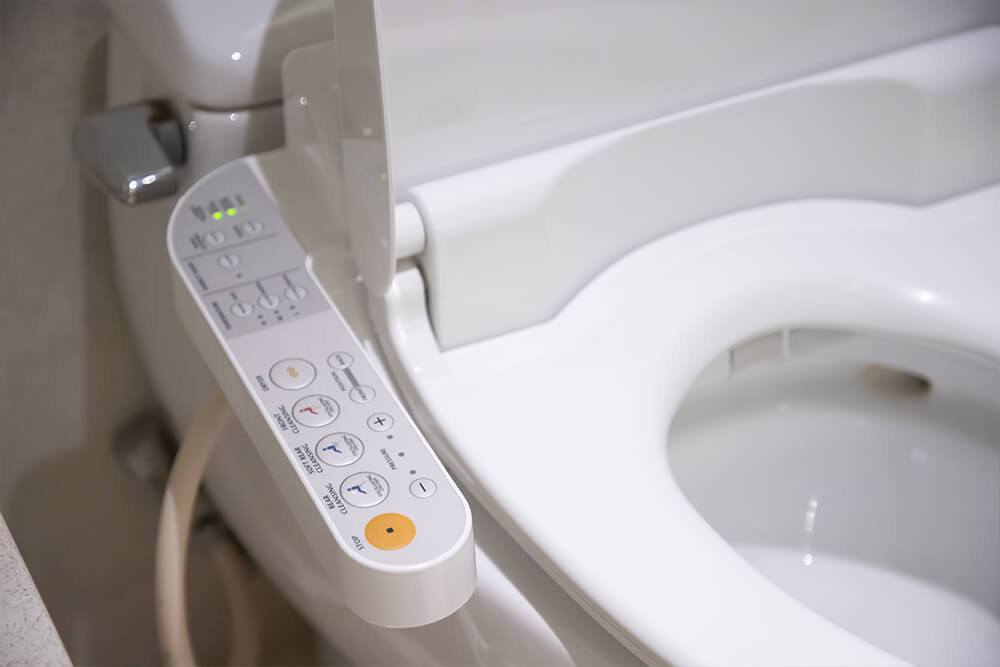The photograph showcases a sophisticated white toilet with an integrated bidet system, primarily highlighting the bidet's complex control panel. The control panel features numerous push buttons, including settings for adjusting the water flow, seat warming, rear cleaning, and soft rear cleansing, among other options that are too blurred to discern clearly. The standout feature is a bright orange stop button that contrasts sharply with the panel's white and light gray tones. The image is centrally focused on the control panel, with a partial view of the toilet seat, bowl, and the connecting hose leading to the water supply. The toilet tank with its silver flush lever is visible but slightly out of focus in the background.